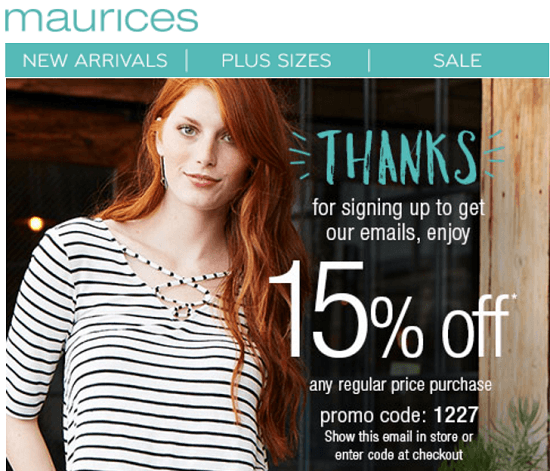This is a promotional screenshot featuring an advertisement for a fashion retailer. The ad highlights several key points:

- **Manicures**, **New Arrivals**, **Plus Sizes**, **Sale** sections.
- An offer of **15% off** any regular-priced purchase with a promo code.
- A "Thanks for signing up" message for subscribing to their emails.

To redeem the discount, customers can either show the email in-store or enter the promo code **1227** at checkout.

In the center of the ad, there is an image of a woman wearing a stylish striped shirt. The shirt features a distinctive lace-up design at the front, with a plunging V-neckline that forms a triangular cut. The shoelace-like ties crisscross over her chest, creating a fashionable and eye-catching detail.

The overall essence of the advertisement is to entice customers with a new seasonal collection, inclusive sizing, and a special discount for email subscribers, while showcasing a trendy, lace-up striped shirt as part of the new arrivals.